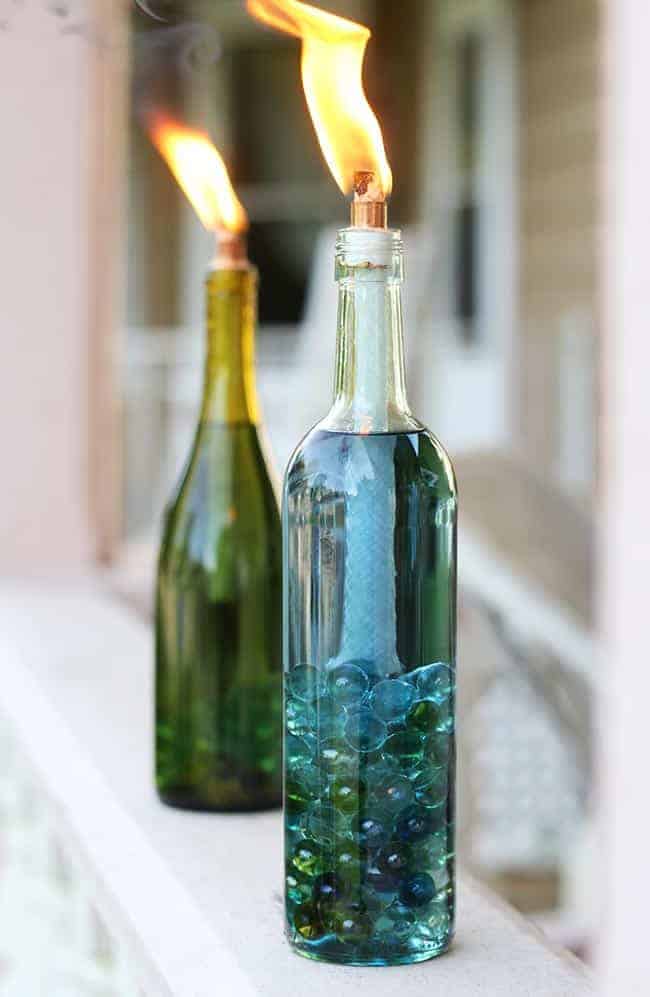The image captures two improvisational lanterns made from wine bottles positioned on a white, shelf-like ledge. The background is a slightly out-of-focus porch area with light brown siding, white window trim, and a hint of a white wicker chair. The bottle on the right, nearest to the viewer, is clear and contains a bluish liquid with an arrangement of clear blue and green marbles at its base. It is topped with a lit wick, resembling a small flaming tiki torch. The flame is a standard orange color with a steady column of smoke. The bottle on the left, positioned further back, is green with a gold top and filled with marbles—though their colors are less discernible due to its distance. This bottle also features a lit wick. Both bottles stand upright on the ledge, casting a warm glow in the sunlight, effectively converting the bottles into makeshift lanterns.